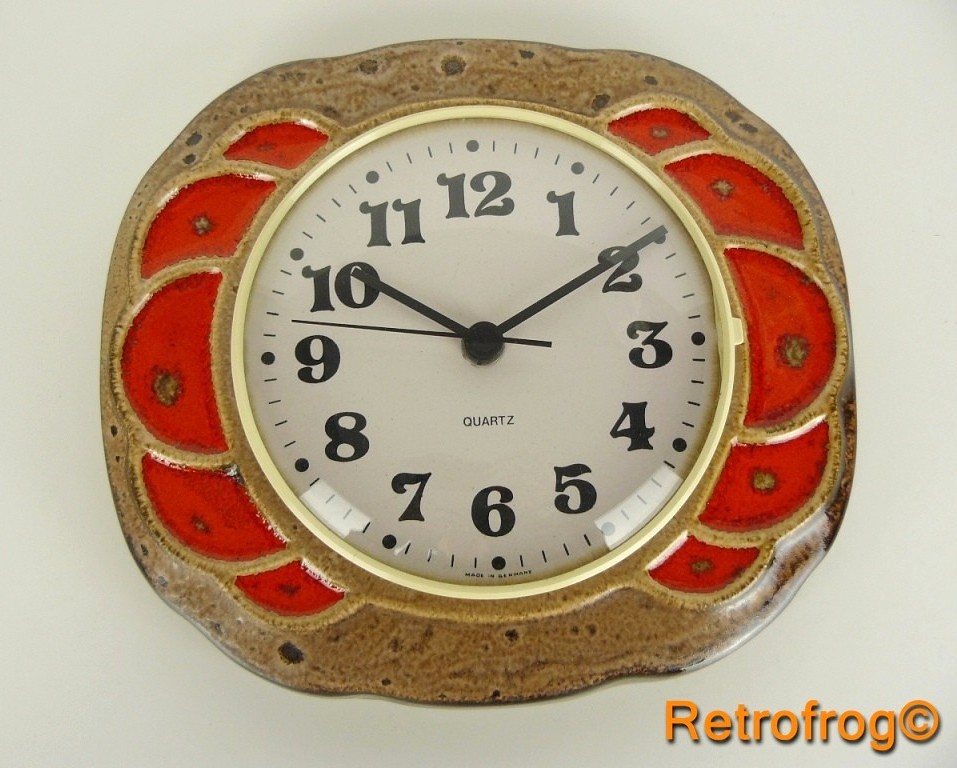The photograph captures an intriguing, vintage-style clock. The clock face, encircled by a gold rim, is white with bold black hands and numerals, prominently displaying the time as 10:10 a.m. and bearing the inscription "Quartz." The clock is set within a distinctive, ornate frame that features a flattened top and bottom, deviating from a perfect circular shape. Surrounding the gold rim are elements reminiscent of red petals, though they do not precisely resemble flower petals, adding to the clock's unique charm. The body of the clock appears to be crafted from a brown material, giving it a rustic, pottery-like or carved rock texture. The overall aesthetic evokes a sense of nostalgia and artistry. At the bottom of the image, the word "RETROFROG" is displayed alongside the copyright symbol.